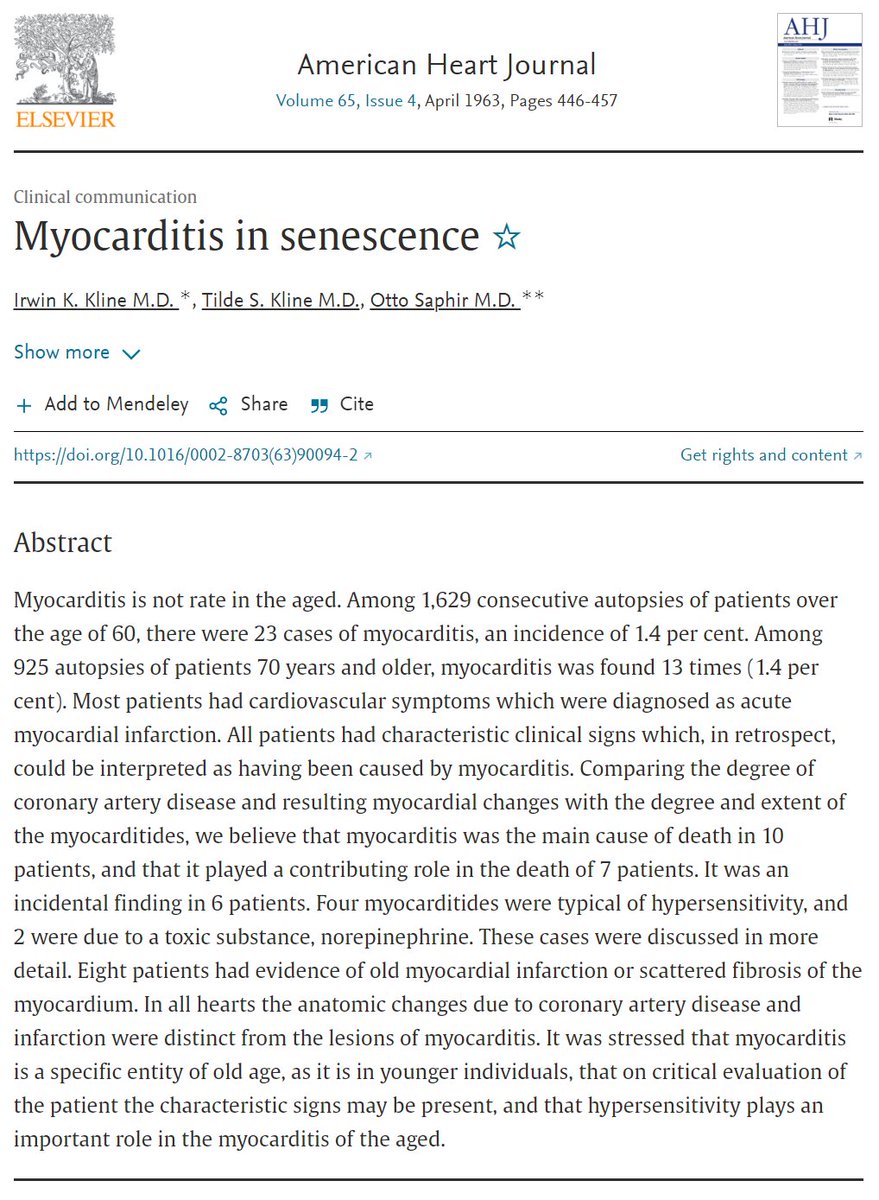The image appears to be a screenshot from a webpage of the "American Heart Journal," published by ELSEVIER. The ELSEVIER logo is prominently displayed at the top in dark yellow, featuring a tree and an owl in white and black. The journal's title, "American Heart Journal," is written in black font with initial capitalization.

Beneath the title, in blue font with initial caps, it says "Volume 65, Issue 4." Further down, in black font, it states "April 1963," followed by "pages 446-457." A horizontal line separates this information from the rest of the content.

Below the line, in gray font, the section is labeled "Clinical Communication." Following that, in larger black font, the title "Myocarditis in Census" is displayed next to an unfilled, blue-outlined star. The authors' names are listed underneath: "Erwin K. Klein, M.D." with an asterisk; "Tilde S. Klein, M.D."; and "Otto Saffer, M.D." with two asterisks. 

Below the authors' names, there is a blue font drop-down menu labeled "Show More." Adjacent to it, a blue plus sign is accompanied by the instruction "Add to Mendeley" in black font with initial caps. There is a blue "Share" button next to the word "Share" in black font, followed by a set of blue quotation marks and the word "Cite" in black.

This detailed description provides a comprehensive visual representation of the webpage screenshot.